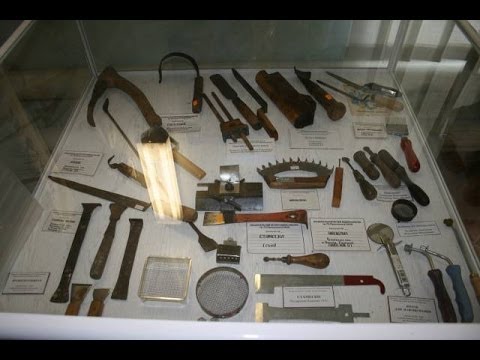The image depicts a photorealistic scene of a museum display case showcasing over 20 vintage tools and farming implements inside a glass enclosure. The tools are arranged on white backdrops, with black-bordered text boxes containing detailed descriptions, which are unfortunately too small to read. At the bottom of the display case, one can find knife-like instruments and a couple of blow torches in the bottom right corner, as well as crowbar-like tools and files in the bottom left. Higher up in the case, there are various indistinct implements, including hook-like tools for grabbing or cutting and a longer, handleless file likely used for cutting. Notably, many of the instruments have rusted over time, indicating their age. The reflection of ceiling lights, caused by the camera flash, is visible in the center-left of the image. In the background, portions of the museum's floor, wall, and a window can be seen, adding context to the setting.